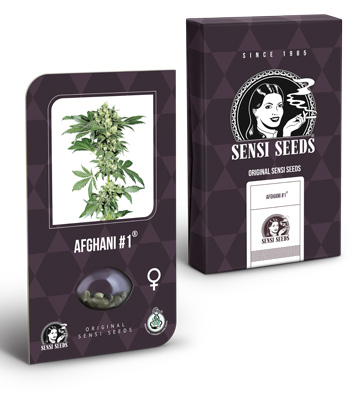The image is a detailed, photographic depiction of a product box set against a completely white background, with shadows adding depth. The main subject is a rectangular, gray box adorned with black hexagonal patterns. Prominently displayed on the box is text that reads "Since 1985" in white, above a black-and-white graphic of a woman smoking a cigarette, encased in a circular design. Beneath this image, the text "Sensi Seeds" and "Original Sensi Seeds" are printed in white. The box features a transparent section revealing the seeds inside.

Adjacent to the main box, there is a depiction of the box's front cover. This cover mirrors the gray and black hexagonal design, featuring the same black-and-white portrait of the woman, with identical text reading "Sensi Seeds" and "Original Sensi Seeds." Adjacent to the cover is a white, rectangular area displaying a green marijuana plant, labeled "Afghani #1." The image builds an impression of a digital recreation of the product packaging, rich in intricate details and coherent in design, emphasizing the branding and heritage of Sensi Seeds.